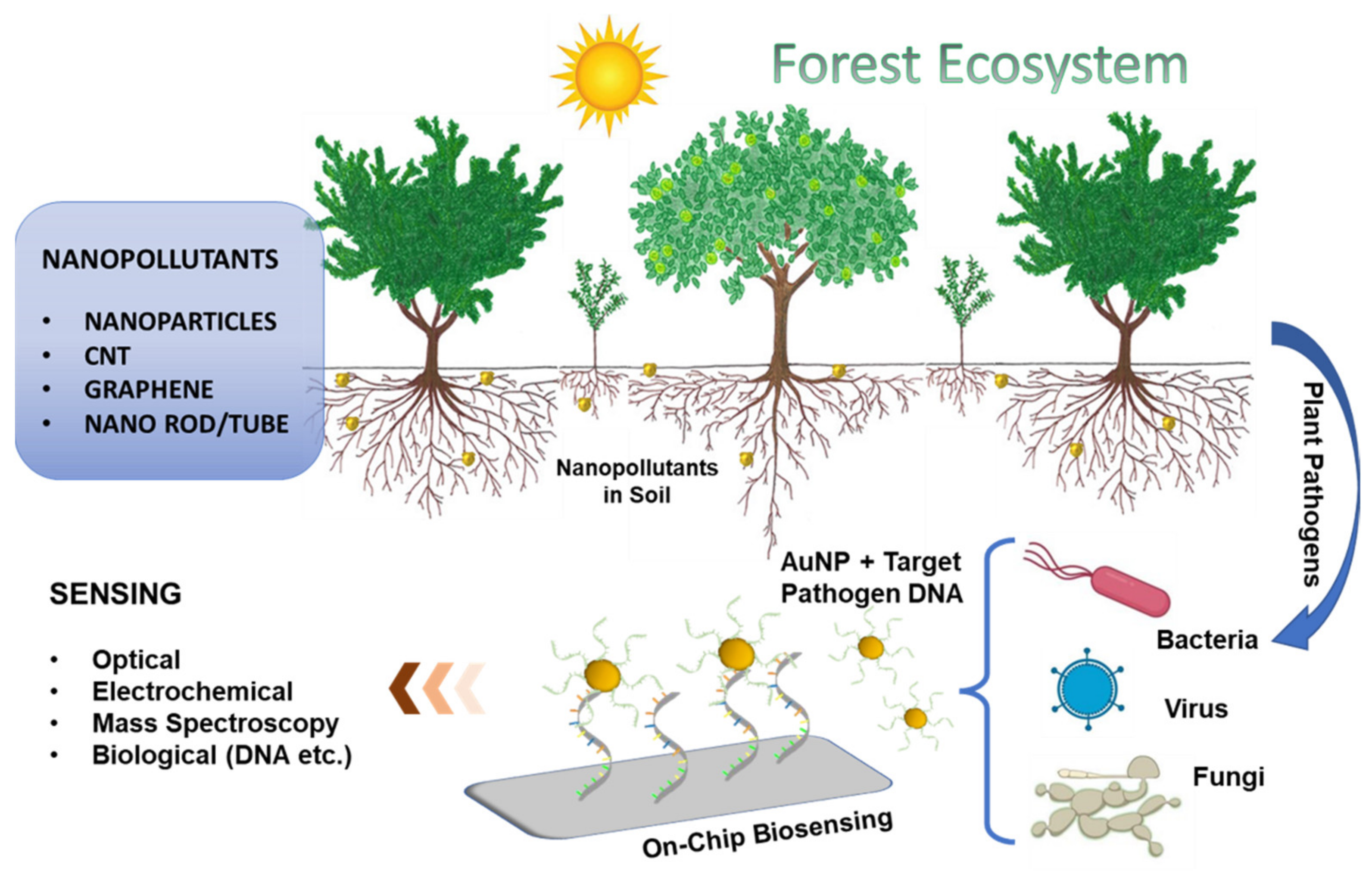The image is a detailed and colorful diagram illustrating a forest ecosystem. At the top of the diagram, the title "Forest Ecosystem" is displayed in green, and a bright yellow sun with radiating rays is positioned in the sky. Three medium-sized trees dominate the top section, with one smaller sapling growing off to the side. Below these trees, a complex network of roots is exposed, showcasing an underground view.

Beneath the soil surface, various informational graphics and arrows provide explanations of the underlying processes. There are text boxes indicating "Nanopollutants," listing items such as nanoparticles, CNT (Carbon Nanotubes), graphene, and nanorods/tubes. Additional text mentions different sensing techniques like optical, electrochemical, mass spectroscopy, and biological methods.

Arrows and labels point to various elements like bacteria, viruses, fungi, and DNA, highlighting their interactions and roles within this ecosystem. A silver panel with yellow bolts, labeled "On-Chip Biosensing," seems to be indicating advanced sensing technology. This intricate diagram seeks to elucidate the complex interactions and impacts of pollutants and pathogens within a forest ecosystem using vibrant graphics and detailed annotations.